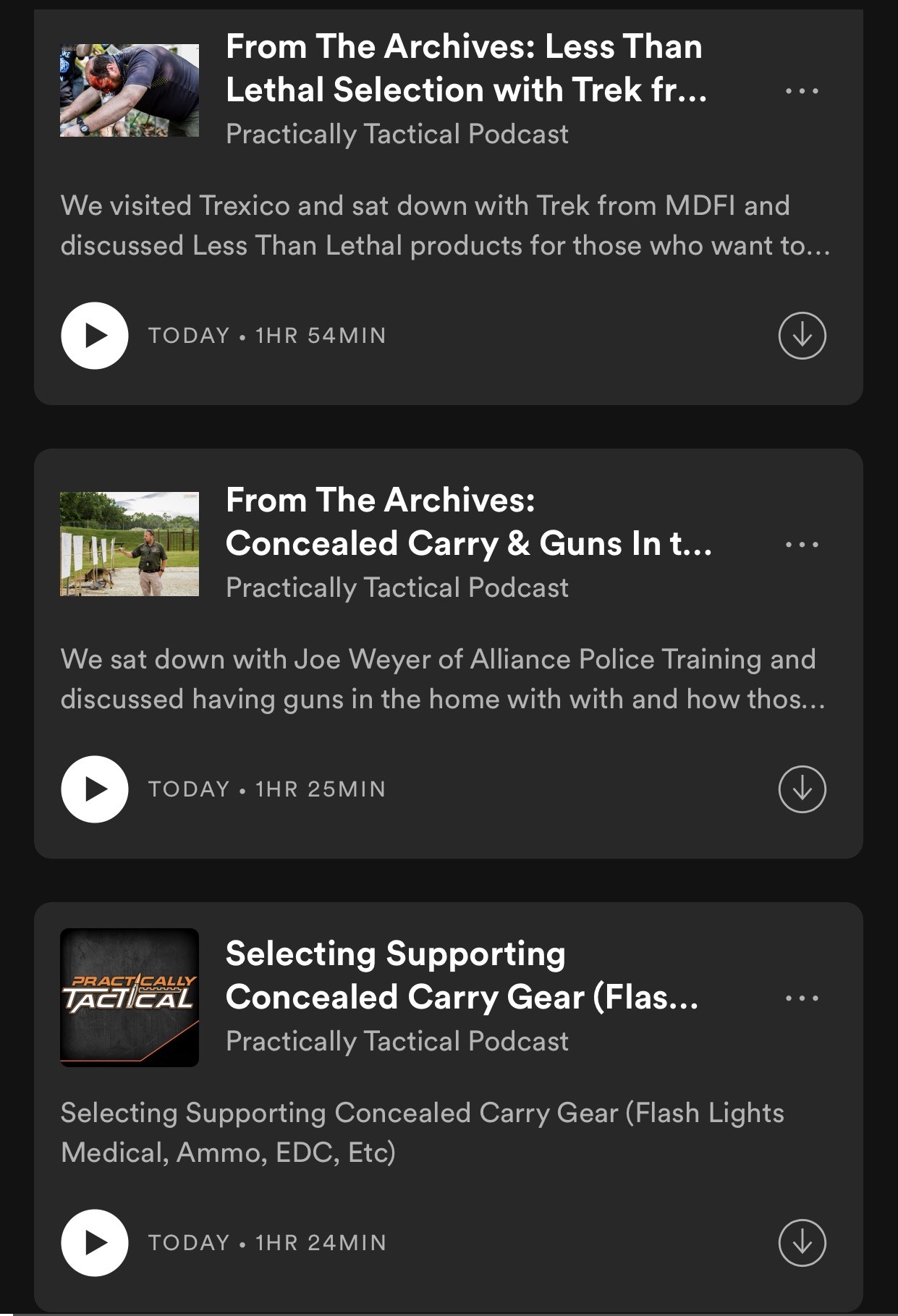The image is a screenshot showcasing a lineup of podcast episodes from the 'Practically Tactical Podcast' series. The podcasts are organized in a vertical list from top to bottom. The first podcast is titled "From the Archives: Less Than Lethal Selection with Trek," followed by visible snippets of the description stating, "We visited Trexaco and sat down with Trek from MDFI and discussed less than lethal products for those who want to..."

The second podcast is titled "From the Archives: Concealed Carry and Guns," with a partial description reading, "We sat down with Joe Ware of Alliance Police Training and discussed having guns in the home with and how those..."

The third and final visible podcast in the list is titled "Selecting Supporting Concealed Carry Gear," with a cut-off description simply stating, "The concealed carry gear...". Despite some truncations, it's evident that each episode provides in-depth discussions centered around various aspects of firearms and personal safety.